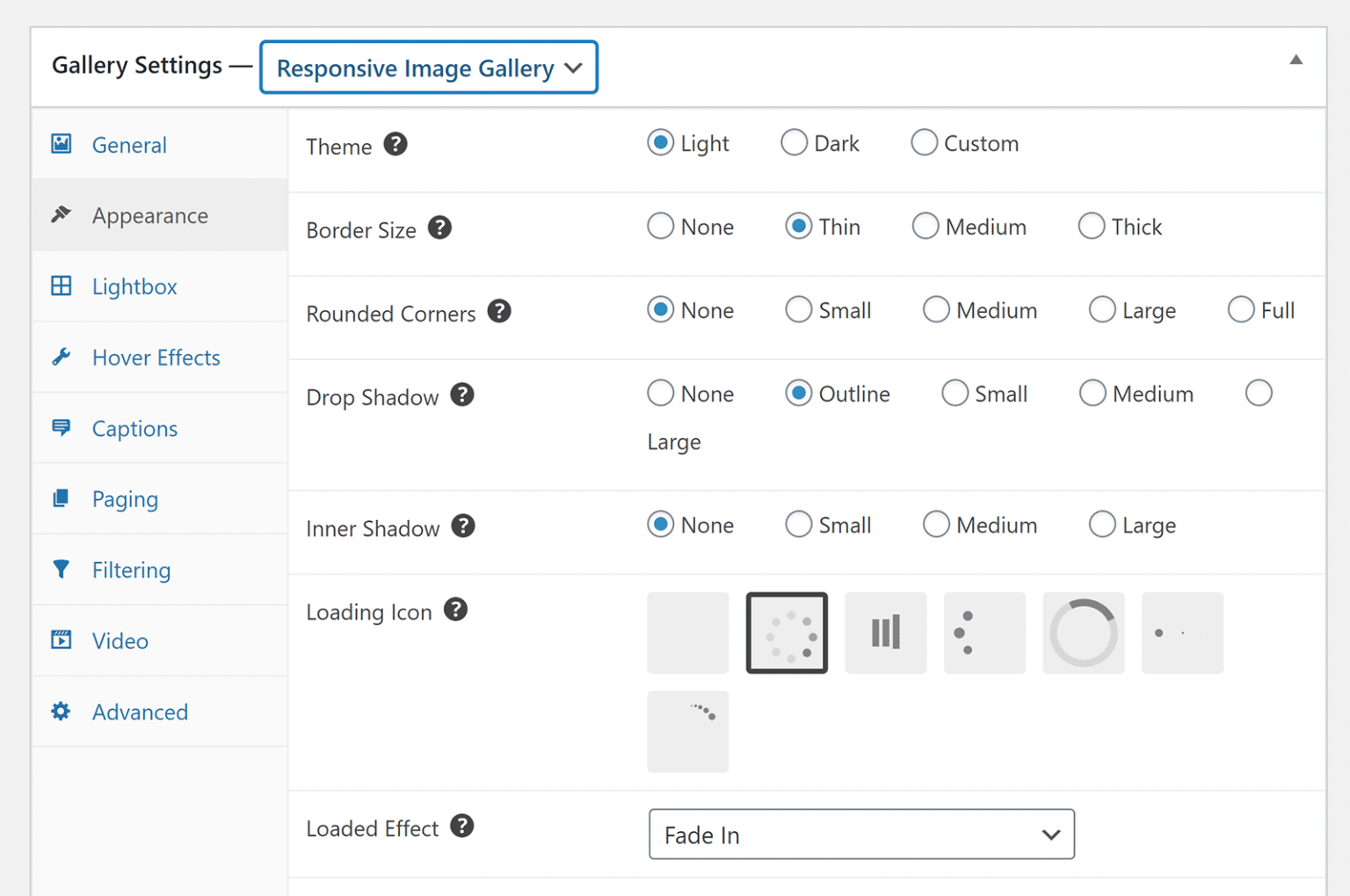This image displays a screenshot from a digital interface, presumably a settings menu for a responsive image gallery tool. The layout is primarily horizontal and is enclosed by a grey border on the top, left, and right sides, with no border at the bottom.

In the upper left corner, the title "Gallery Settings" is prominently displayed in bold black text. Adjacent to this, within a blue rectangular box, is the text "Responsive Image Gallery" accompanied by a down arrow indicating a dropdown menu for more options.

On the left-hand side of the screen, a vertical menu lists various options, each prefaced by an icon. The highlighted option, "Appearance," is shown in black, signifying it is the current selection. The other options, displayed in blue, include "General," "Lightbox," "Hover Effects," "Captions," "Paging," "Filtering," "Video," and "Advanced."

To the right of this menu, a series of configurable settings are presented in black text. Each setting is associated with a black circle containing a white question mark, indicating help or additional information is available. These settings include:
- Theme: with selectable options "Light" (highlighted), "Dark," and "Custom."
- Border Size: selectable options "None," "Thin" (highlighted), "Medium," and "Thick."
- Rounded Corners: not specifically detailed in the given content.
- Drop Shadow: selectable options "None" (highlighted), "Small," "Medium," "Large."
- Inner Shadow: selectable options "None," "Outline" (highlighted), "Small," "Medium," "Large."
- Loading Icon: a specific icon has been chosen, though not detailed.
- Loaded Effect: the chosen option is "Fade In."

This concluded description provides a thorough representation of the screenshot's layout and contents, detailing the options and selections available within this responsive image gallery setting interface.